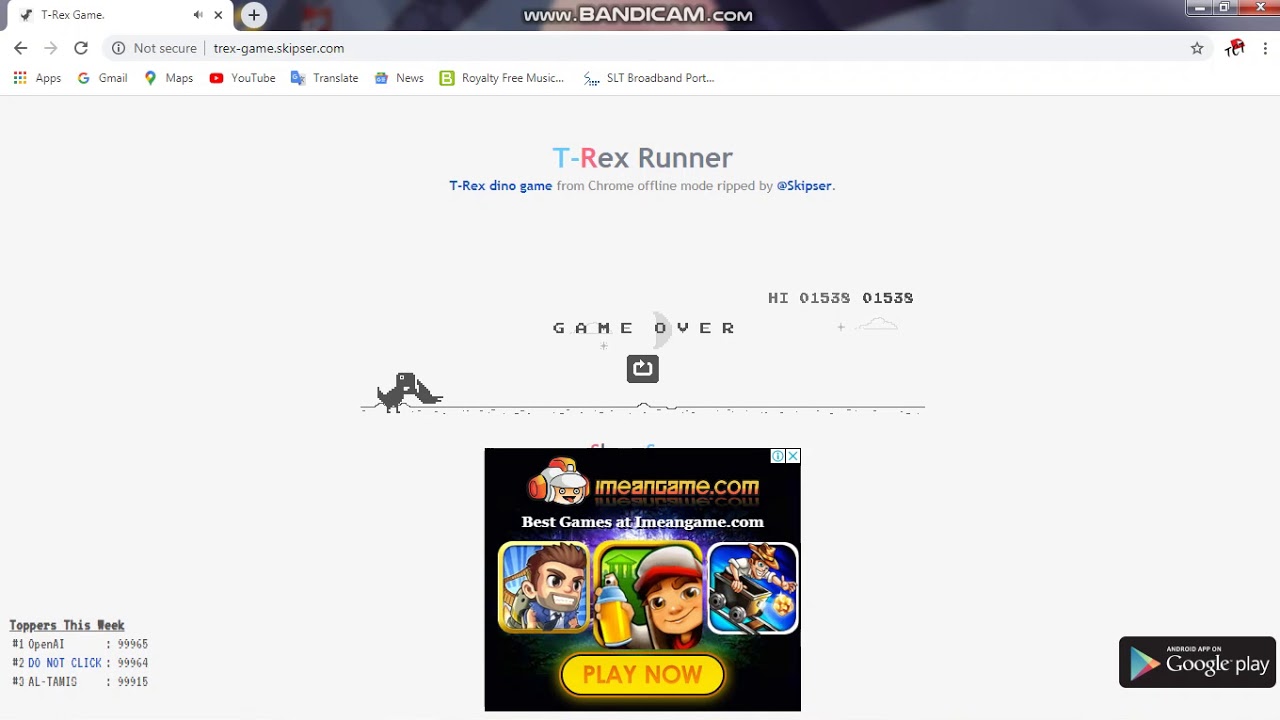This image is a detailed screenshot of a web browser displaying a game page. The top banner is a mix of gray, black, and red, with white text prominently displaying the URL "www.bandicam.com" at the center. On the left of the screen, there is an open tab labeled "T-Rex Game" in black text on a white background, accompanied by an illustrated black T-Rex.

Directly below the banner is an address bar containing the URL "trexgame.skipzer.com." Central to the webpage is the title "T-Rex Runner, T-Rex Dino Game from Chrome offline mode ripped at skipser." Beneath this title, the screen shows a score labeled "High 1538," followed by the text "Game Over."

Towards the bottom of the screen is a black square graphic with cartoon-like characters and the text "I mean game.com." A yellow button on this square prominently features the prompt "Play Now."